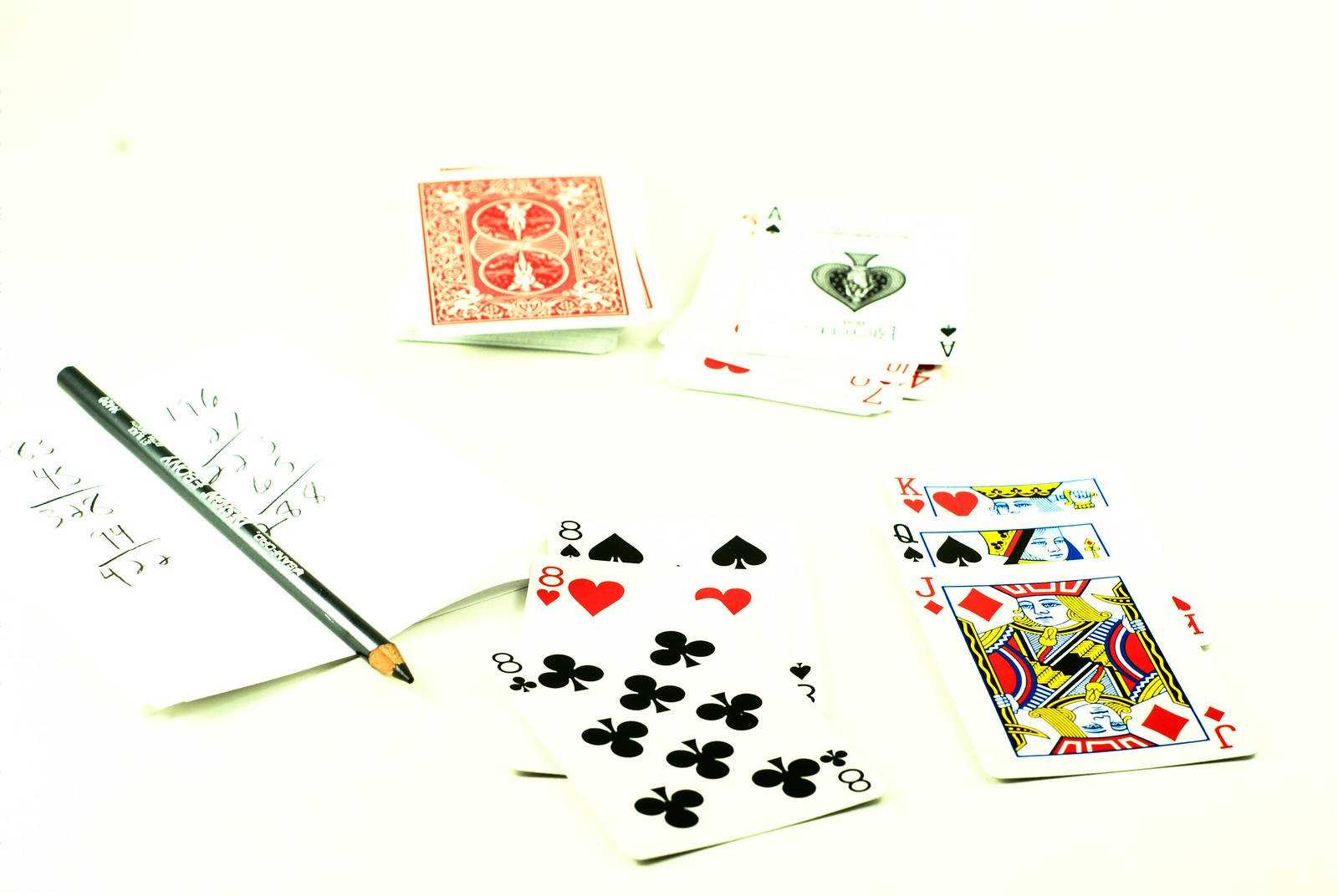In this image of a card game in progress, the central focus is on a neat stack of three eights: the eight of spades, the eight of hearts, and the eight of clubs. The eight of clubs, tilted slightly to the right, crowns the pile. Nearby, a player’s hand is visible, holding the king of hearts, the queen of spades, and the jack of diamonds. Above this hand, a draw pile of ornately designed red-backed cards with three central circles—two dark red and one light red—awaits the next turn. To the left of the main play area is a discard pile topped with the ace of spades.

Off to the side, a score sheet holds the tally for two players. The scores, written in black pencil, read as 288 for one player and 422 for the other. The sharpened, eraser-less pencil rests between the two columns of scores, indicating a game that has been closely tracked and intensely played. The scene captures a moment of strategy and suspense, with every detail in place for a riveting card game.